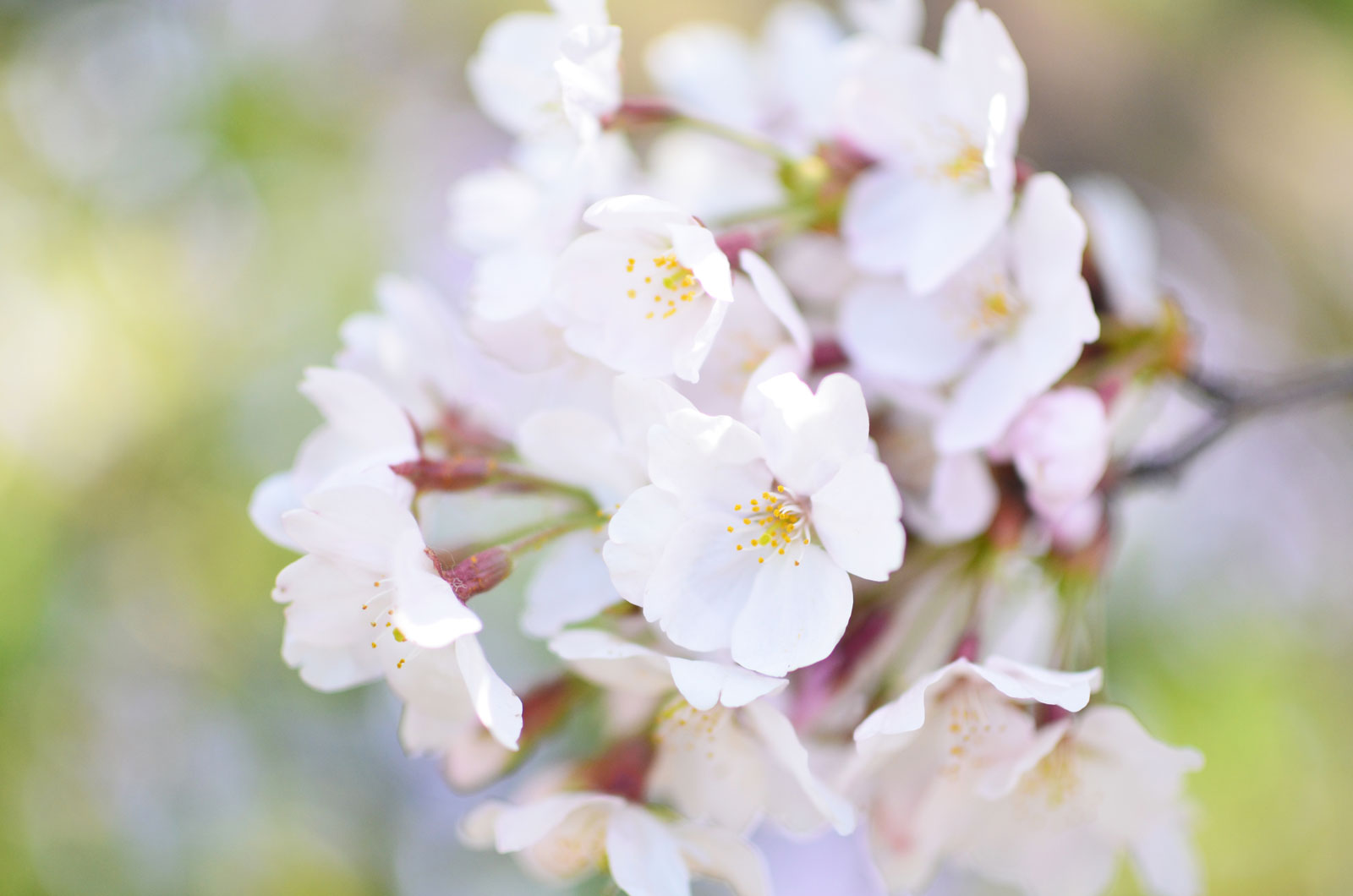The photograph is a close-up, portrait-mode image of a flower, emphasizing its intricate details while blurring out the outdoor background of greens and whites to create a soft focus. Centered in the image, the flower, consisting of tiny white florets with six heart-shaped petals, forms a composite bloom. Each small flower reveals a yellow stamen, hinting at pollen. The central head of the flower is turned to the left side of the picture. The green stems supporting the blooms exhibit subtle purple tinges at their tips. No text indicates the flower type, and the absence of additional elements keeps the focus solely on the delicate, multi-petaled flower against the blurred backdrop.